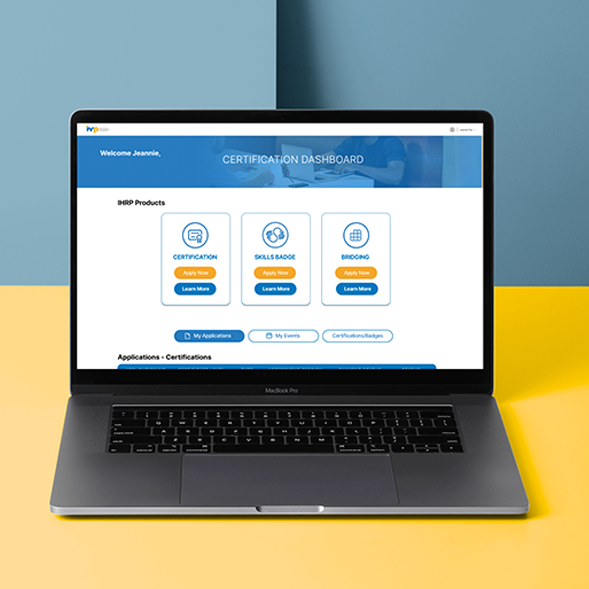The image showcases a MacBook Pro positioned on a yellow desk or table, set against a blue wall with an indented section, casting a subtle shadow. The laptop itself sports a sleek gray finish and features a black keyboard. Open on the laptop screen is a webpage displayed under the title "Welcome Genie," labeled as a "Certification Dashboard." The page prominently features a banner displaying an image of two individuals seated across from each other at a table; one is using a white laptop and wears a blue t-shirt while typing. Below the banner, the computer screen is divided into three rectangular boxes labeled "Certification," "Skills Badge," and an indistinguishable third label. Each box has an orange "Apply Now" button followed by a blue "Learn More" button underneath. Additionally, there are three oval buttons beneath these boxes, labeled "My Application," "My Events," and an unreadable third option.